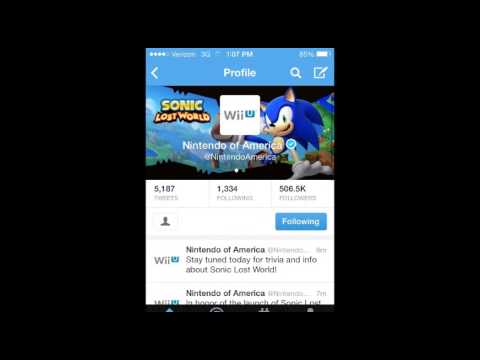The image is a screenshot presented within a large black rectangle, set against a black background in a landscape orientation. At the heart of the screenshot is a cell phone display showcasing information related to Sonic Lost World, a game associated with the Wii U, featuring an image of Sonic the Hedgehog, the iconic blue character.

The top of the cell phone screen is adorned with a blue band. In the top left corner, there are four filled circles along with the text "Verizon." The time is indistinct due to blurriness, but the battery icon shows a full charge. Centered within the blue band is the word "profile" in white text.

Beneath the blue band, there is a graphic dominated by vibrant colors. On the right side of the graphic, the text "Sonic Lost World" is displayed in bold yellow against a blue backdrop beside an image of Sonic the Hedgehog. They collectively present a cartoonish landscape scene. Within this graphic, there is a white rectangle containing the word "Wii U" in gray and teal lettering, respectively.

Below this main graphic, the screen shows more detailed information. On the left side, a statistic box reveals "5,187" tweets, though the text is partially blurry. The center statistic box shows "1,334 followers," and to the right, another box lists "506.5K" followers, though it is slightly unclear.

Adjacent to these statistics, there is an icon of a person inside a box, followed by a blue rectangular "Following" button with white text ensuring visibility.

The section beneath contains the Wii U and Nintendo of America logos, and it reads "Stay tuned today for trivia and info about Sonic Lost World."

Finally, there is additional information from Nintendo of America, beginning with the phrase, "In honor of the launch of Sonic Lost," before the text gets cut off, ending the visible portion of the screenshot.